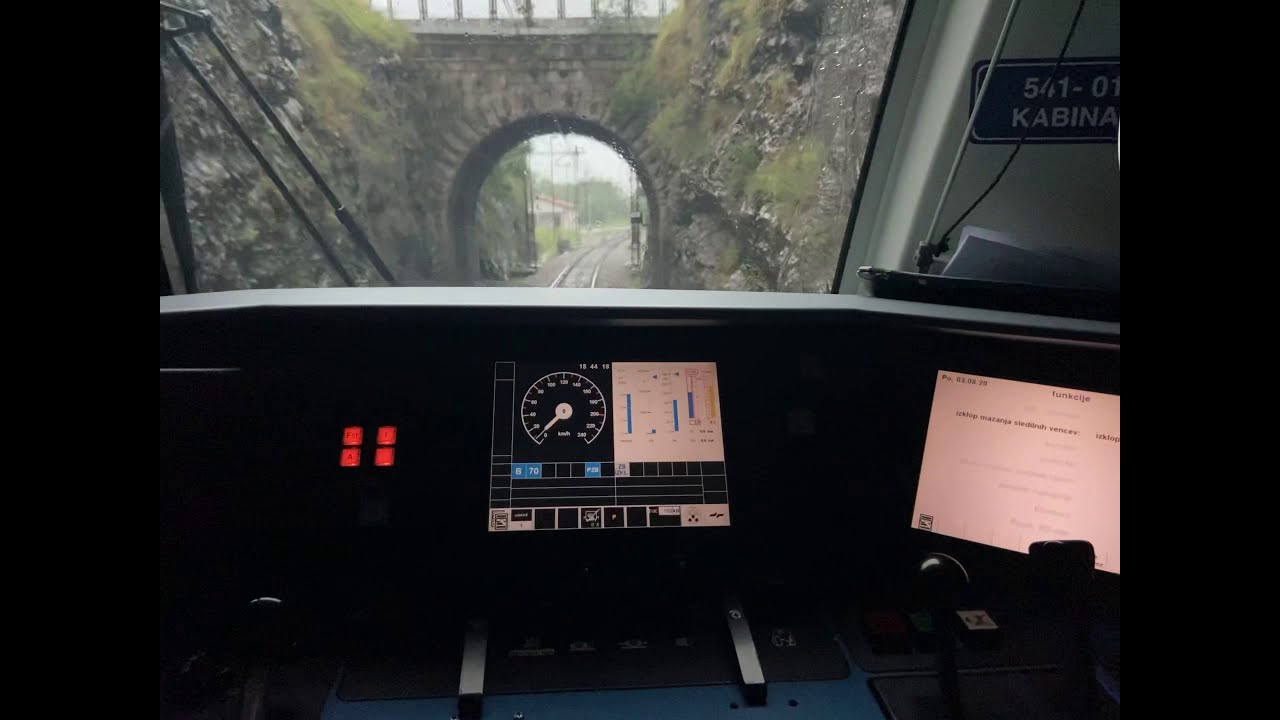The photograph captures the view from inside the driver's cabin of a train. The bottom section prominently features the instrument panel, which includes a central black square displaying a speedometer, and a white square with various informational displays, such as graphs and charts. Adjacent to it are illuminated red dots and blue dots on a black chart. To the far right, a tilted white screen is visible. Looking out through the front windshield, the train is about to pass through an arched bridge made of brown-colored bricks, flanked by solid rock walls. The arch leads to a scene of distant railroad tracks, power lines, trees, and a building slightly to the left. A sticker in the upper right corner of the windshield reads "501-01 K-A-B-I-N-A" in white text on a blue background. Above the arch, the bridge acts as a walkway crossing over the tracks. The setting is framed by a cavernous landscape and a gray sky overhead.